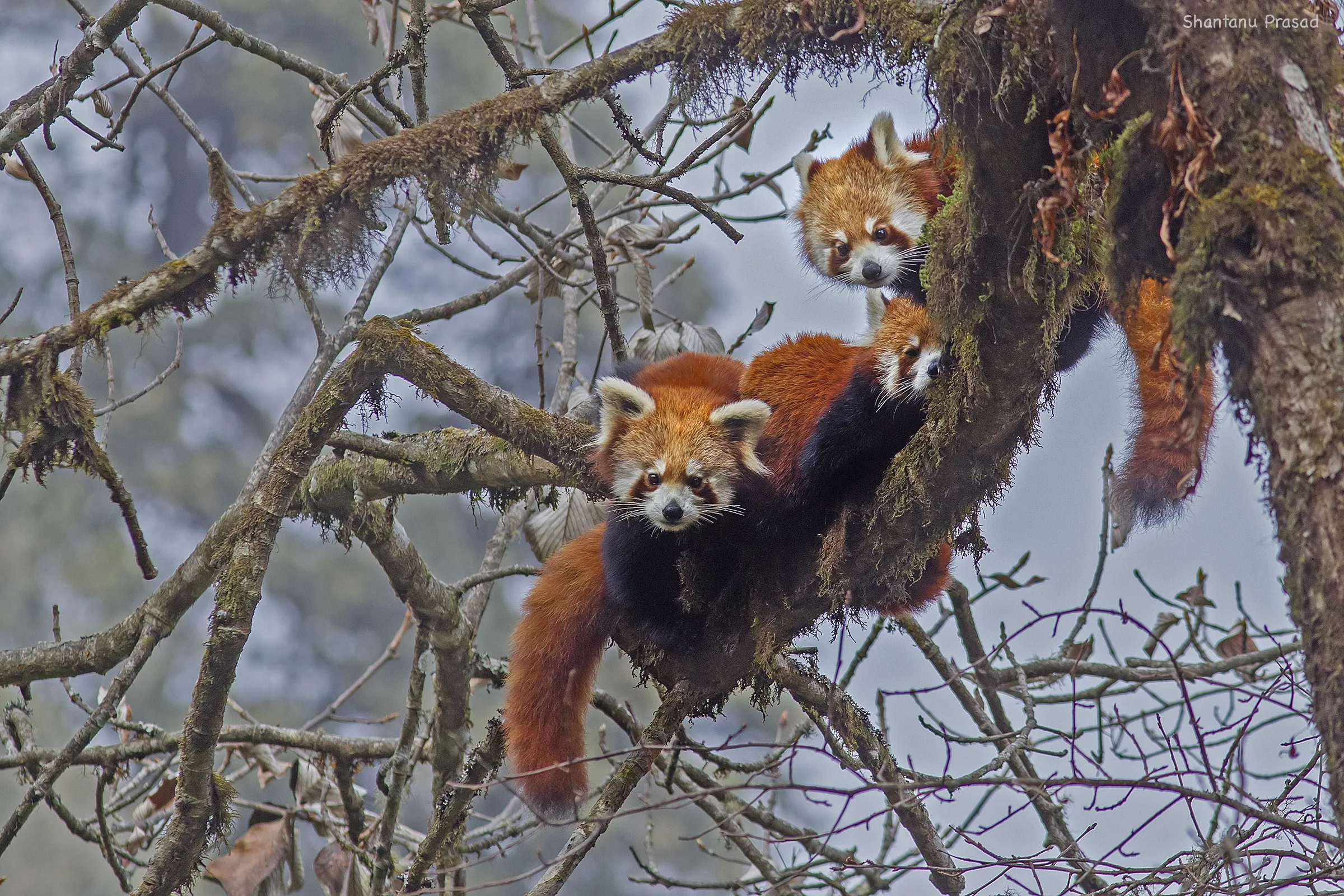In this detailed photograph taken by Shantou Prasad, three red pandas are perched in a bare, moss-covered tree on a cold winter's day. The tree, devoid of leaves and showing signs of frost amidst a few scattered brown leaves, serves as an intriguing backdrop for these curious creatures. The pandas are reddish-brown with lighter brown faces that are distinctively bordered with white markings. Their features include black rings around their eyes, a black nose, whiskers, and pointed white ears. The foreground shows two pandas gazing directly at the camera, their expressions seemingly inquisitive. One is fully visible, displaying his black eyes and bushy red tail, while another lies along a branch, his face half-obscured by the mossy limb, appearing less engaged. The third panda peeks from behind the branch, adding a playful element to the scene. The composition captures the pandas in their natural habitat, seemingly curious about the viewer’s presence.